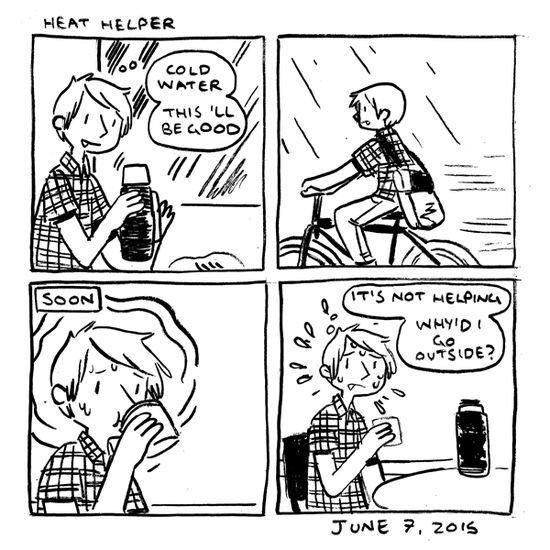The image is a four-panel black and white cartoon strip titled "Heat Helper." In the top-left panel, a young man in a plaid shirt is capping a thermos with a black base and white top, thinking, "Cold water, this'll be good." In the top-right panel, the same young man is riding a bicycle in the rain, moving leftward with raindrops indicated by small lines. In the bottom-left panel, marked "Soon," the young man is sitting down, drinking from the thermos cap, with beads of sweat on his face. The final bottom-right panel shows the man still seated, sweating profusely and lamenting, "It's not helping, why'd I go outside?" Beneath this panel, outside the comic strip, the date "June 7, 2015" is written in black.